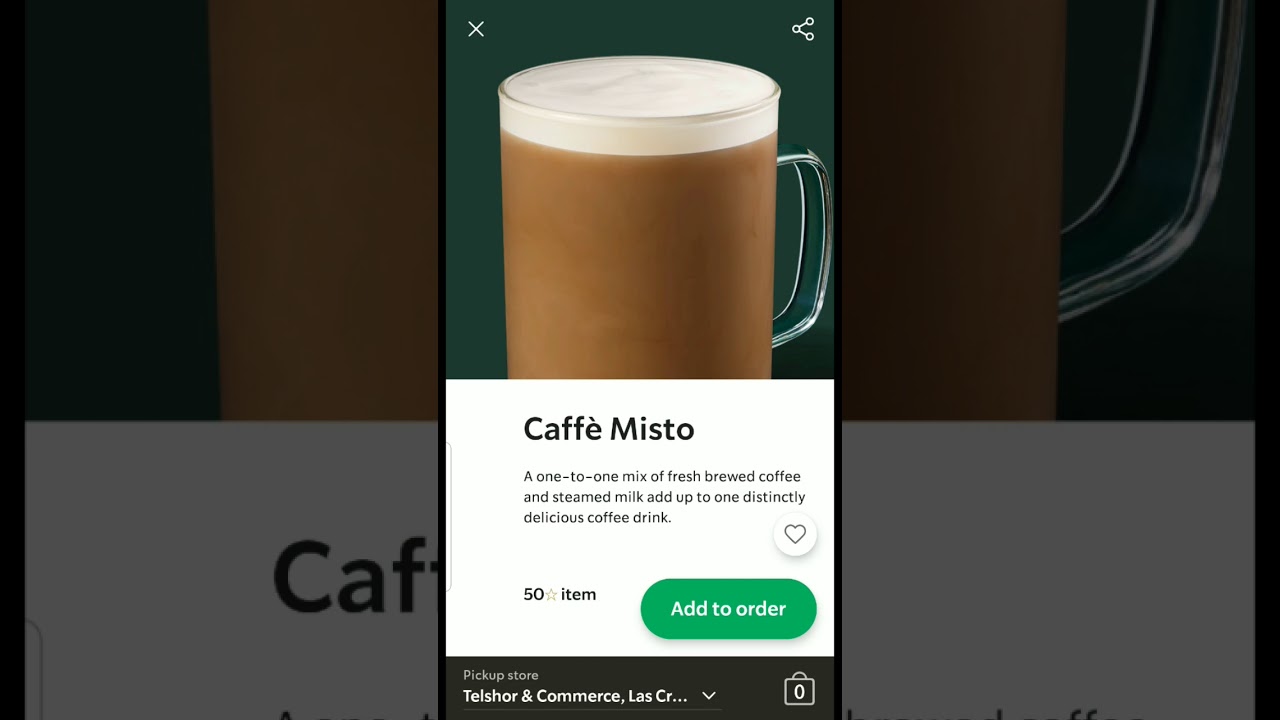The image features a prominently displayed, large coffee mug filled with rich, brown coffee. The setting is a notably dark-themed website, which emphasizes the contrasting bright elements of the coffee cup. The mug, which also includes a transparent glass handle, is identical to the one highlighted by a pop-up overlay on the same page. 

The pop-up provides additional clarity and details: it introduces the drink as "Café Misto," suggesting a blend of freshly brewed coffee and steamed milk. The text within the pop-up is situated in a white box, which visually stands out against the dark background, and states, "Café Misto: a one-to-one mix of fresh brewed coffee and steamed milk adds up to one distinctly delicious coffee drink."

Additional elements in the pop-up include:
- A button to add the item to an order, priced at $50.
- Interactive icons, such as a heart for 'liking' and options for sharing, indicating a focus on taste, sharing, and e-commerce.
- A partially visible text at the bottom indicating there might be more information cut off by the pop-up.

To the left of the coffee mug image within the pop-up, there are icons, including what appears to be a shopping bag. Part of the text in the background image is obscured by the pop-up but hints at the letters “CAF,” presumably part of the website's branding.